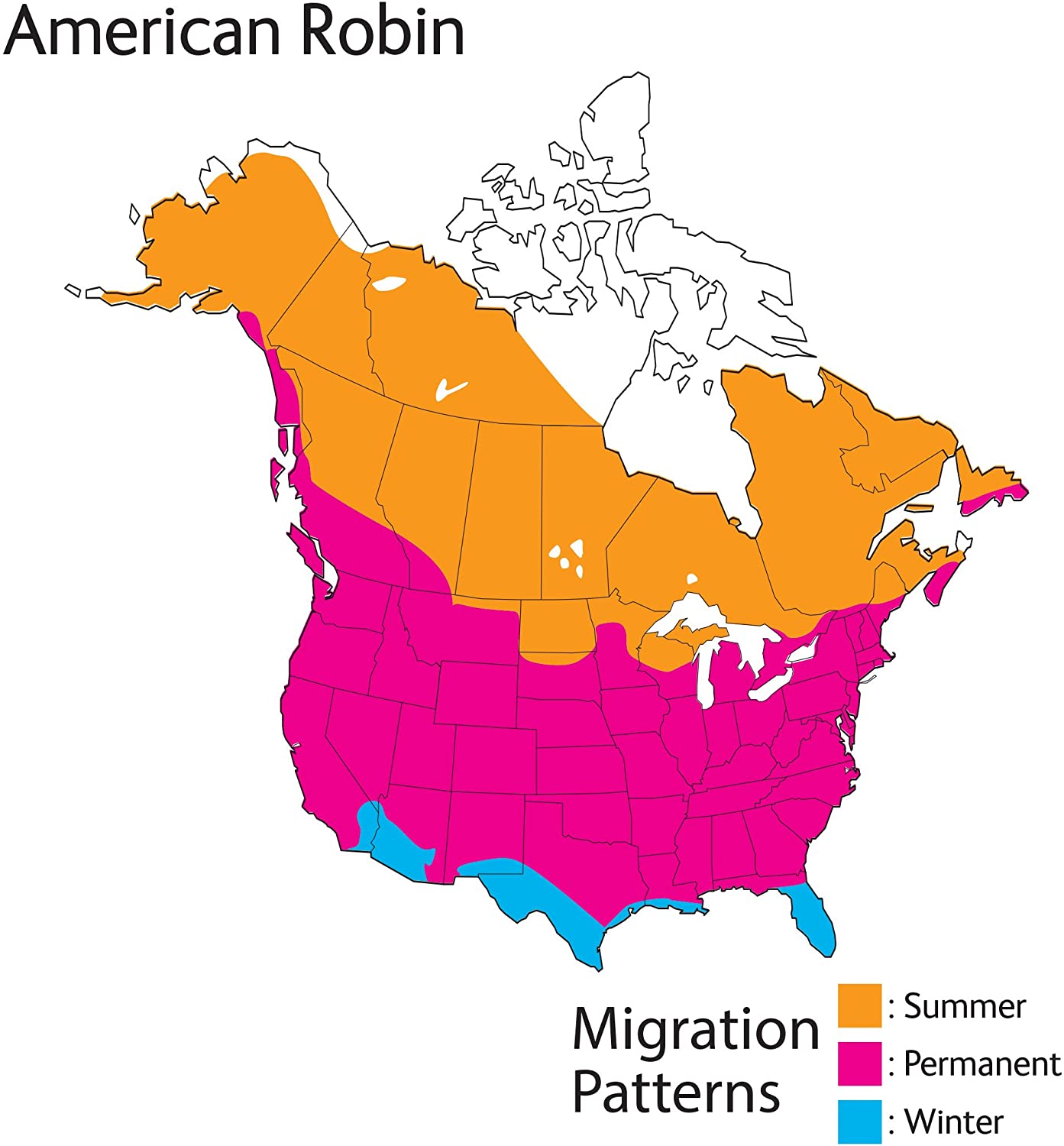The image displays a detailed colored map of the North American Hemisphere, specifically highlighting the United States, Canada, and Alaska. The title "Migration Patterns" is prominently shown in black print on a white background beneath the map. To the right, three color-coded blocks are present: the top block is orange labeled "summer," the middle block is magenta labeled "permanent," and the bottom block is blue labeled "winter." These color blocks correspond to the regions on the map, indicating the American Robin's migration patterns. The orange regions, mostly encompassing Canada and Alaska, signify their summer habitats. The magenta regions cover the majority of the United States and parts of Canada, representing their permanent habitats. The blue regions, which include the southern parts of the United States such as parts of Florida, Texas, New Mexico, and sections of California and Nevada, denote their winter habitats. This detailed depiction illustrates where the American Robins migrate throughout the year: summers in the upper parts of Canada and Alaska, permanent residence primarily in the United States, and winters in the southern states.